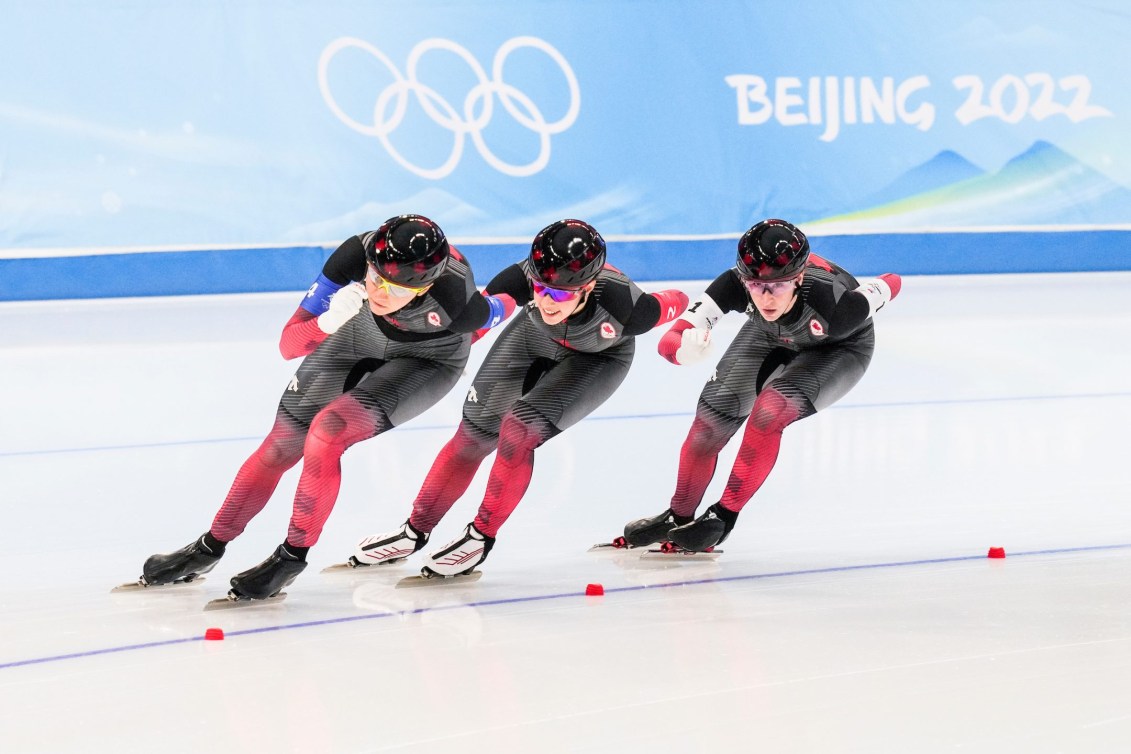The photograph captures a vibrant moment from the Beijing 2022 Winter Olympics, showcasing three Canadian speed skaters in a dynamic formation, gliding in unison on a curved ice track. The backdrop features a clear blue sky and a picturesque mountain range, adorned with the Olympic rings and the text "Beijing 2022" prominently displayed. Each skater dons a sleek, skin-tight uniform with a black torso and red shins and forearms, all emblazoned with the iconic maple leaf of Canada. Their helmets are uniformly black, adorned with the red maple leaf, and their protective eyewear varies in color and style – one with yellow-rimmed glasses, another with purple and pink, and the last with clear lenses. The skaters have distinctive numbers on their arms – four, two, and one – and their skates are different shades: the front and rear athletes wear black skates, while the central skater sports white skates with red accents. Bent over in intense focus, the trio speeds gracefully across the ice, epitomizing Olympic spirit and national pride.